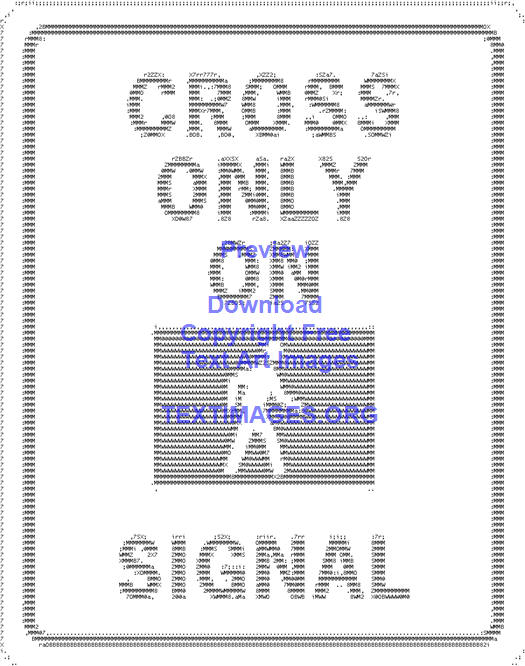The image depicts a sign with a white background, featuring the bold, uppercase instruction "CROSS ONLY ON SIGNAL." This text is bordered by an intricate design created entirely from typewriter or keyboard characters. A highlighted black box spans the space between the words "ON" and "SIGNAL", containing a pixelated, yet distinctly recognizable, white silhouette of a pedestrian mid-stride—crafted meticulously by leaving blank spaces where needed to form the shape. Overlaid on the sign is text in blue and purple, some in mixed-case: "Preview", "Download", "Copyright-free", "Text Art Images", and "TEXTIMAGES.ORG". The website mentioned, textimages.org, offers more of these unique text-based art pieces.